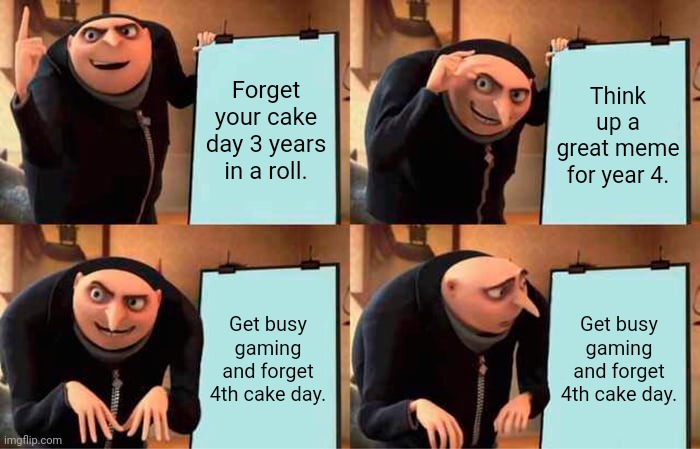A humorous multi-panel meme featuring a hunchbacked man dressed in a black, long-sleeve outfit with a front zipper. In the top left panel, he points a finger upwards, accompanied by a piece of paper reading, "Forget your cake day three years in a row." In the top right panel, he holds his finger and thumb close together, as if indicating something tiny, next to a poster board with a light blue background and black text that says, "Think up a great name for year four."

In the bottom left panel, the man is hunched over, pointing towards the ground with his fingertips nearly touching the floor, beside a piece of paper that reads, "Get busy gaming and forget fourth cake day." The bottom left corner of this panel features the watermark "IMGflip.com" in white writing. Finally, in the bottom right panel, the man appears stressed, staring at a piece of paper with the same message, "Get busy gaming and forget fourth cake day," as he continues to point towards the ground.